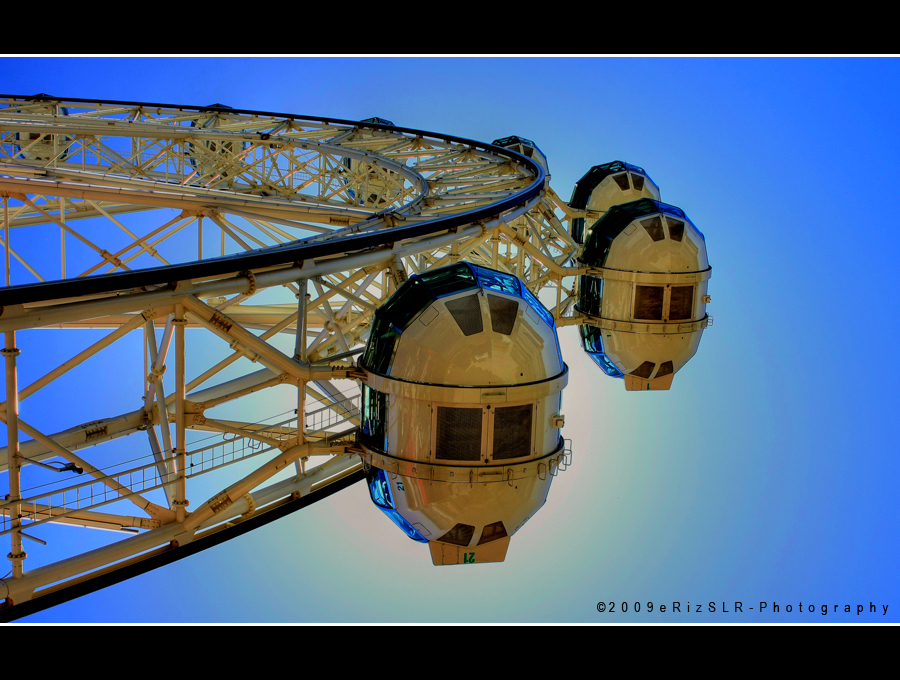The image is a color photograph in landscape format, presented in a widescreen movie-like style with black horizontal strips at the top and bottom. Thin white lines separate these black strips from the main image, framing it elegantly. The photograph appears to be professionally taken, evidenced by a copyright marking in the bottom right corner, reading "© 2009 eRiz SLR-Photography."

The photograph captures a Ferris wheel from a unique, upward-looking perspective, as if viewed from directly below but slightly in front. The Ferris wheel, constructed predominantly of white metal with a black piping rim around its circumference, extends upwards into a brilliant blue sky. Notably, only the right half of the Ferris wheel is visible, as the left half extends out of frame, creating a striking semicircular composition.

Each of the seven visible pods, or capsules, attached to the wheel, features a distinctive design, being enclosed with black and white sections and windows, contrasting with the traditional open swing seats. The overall structure of the wheel includes metal rods forming the framework, with brown edges contributing to its intricate appearance.